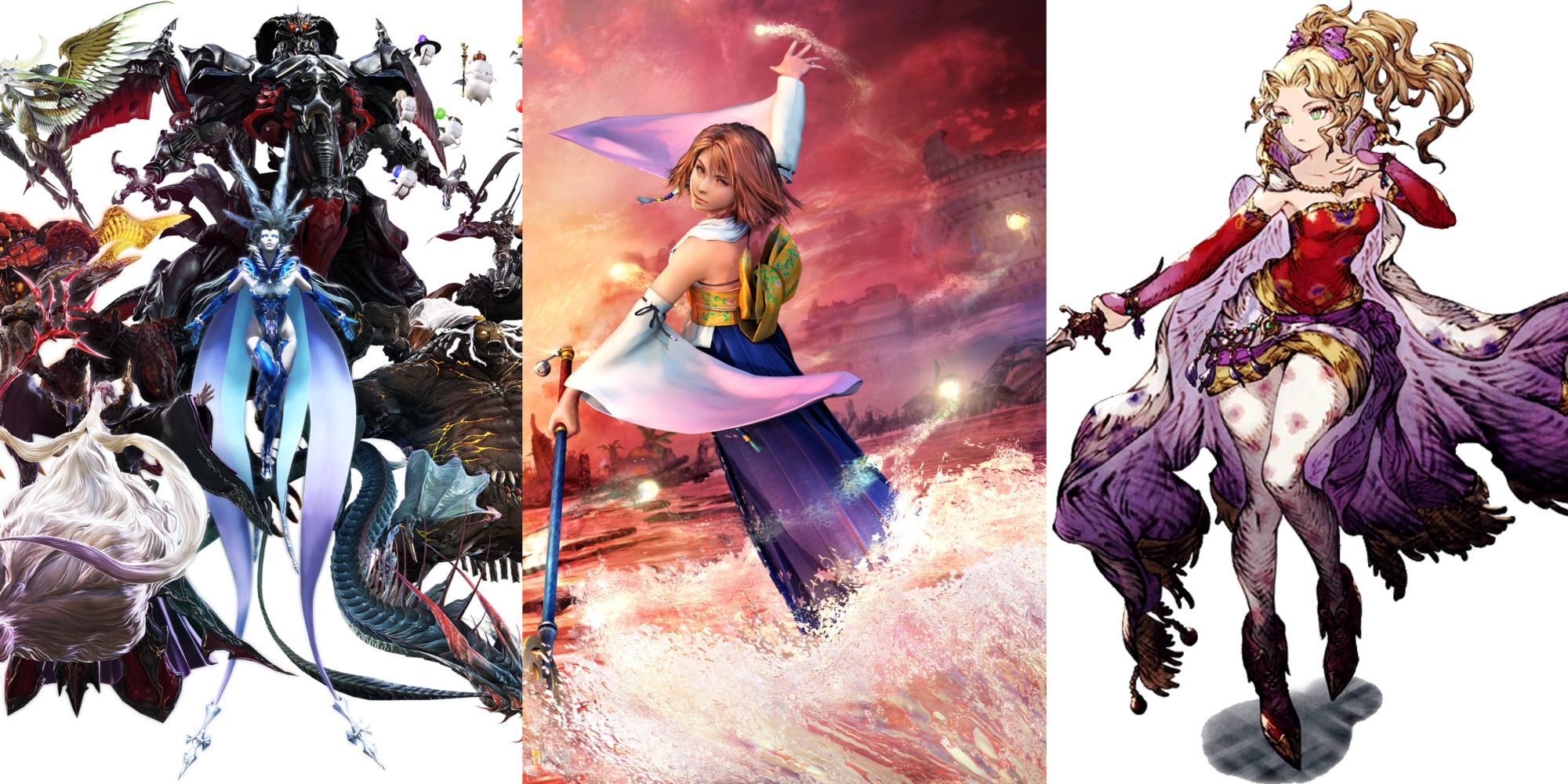This composition features three side-by-side, anime or manga-style illustrations of female characters, each set in their distinct fantasy environment. On the far left, a formidable, alien-like figure clad in blue commands attention with spikes protruding from her head and expansive blue wings. She is surrounded by a host of fantastical creatures, including a serpentine dragon, a monstrous figure adorned in red and black, and whimsical, marshmallow-like beings with tiny hats.

In the middle image, a young woman stands powerfully in tumultuous waters against a stormy, blood-red backdrop. She wields a staff-like weapon and is adorned in elaborate attire consisting of long, flowing white and purple sleeves, a yellow top, and a purple skirt. Her scene is marked by a sense of impending chaos and action, heightened by the dramatic, dark waves at her feet.

On the far right, a character reminiscent of a pirate princess with flowing blonde hair appears to be in mid-motion, perhaps engaged in battle. She is attired in a striking ensemble that includes a red bodice, a short yellow skirt, and a flowing purple cape. She clutches a sword, ready for action, her white boots emblazoned with floral designs adding a touch of elegance to her combat-ready stance.